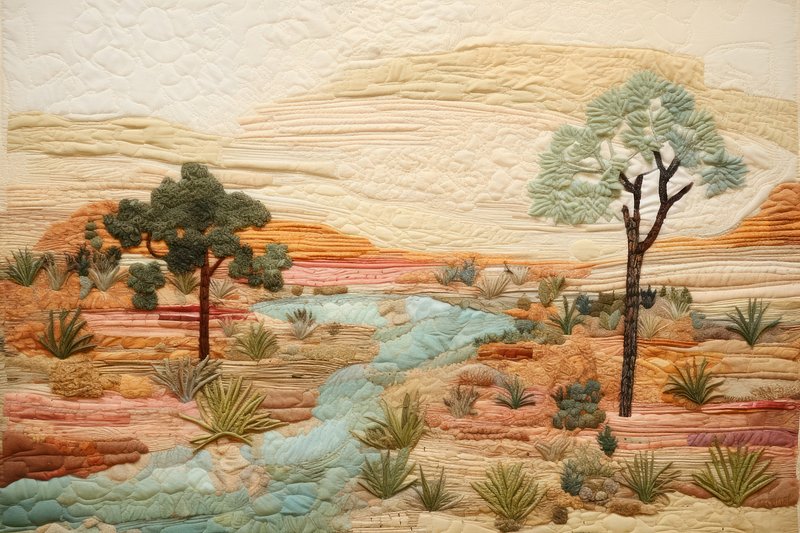The image captures a desert oasis in exquisite detail, possibly portrayed in a painting with raised elements, adding to its textured and tactile quality. At the center of the composition is a light blue creek, flowing through the middle, culminating in a pool and looping back upon itself. On the left side, a vibrant tree is surrounded by an array of plants, including cacti, with various hues of green, cyan, orange, and red interspersed at its base. The creek cuts through a dynamic landscape, set against a visually striking backdrop of red, orange, maroon, and beige shades, reflecting rugged desert rocks and dunes. The entire scene merges seamlessly with a tan and white background, which exhibits a depressed texture reminiscent of stone scales commonly found in such arid regions. The right side mirrors this botanical diversity but features a taller, light green tree with a brown base, enhancing the visual balance of the scene. The sky, depicted in muted white and beige tones, completes the depiction, hinting at either distant mountains or just the vast desert horizon. This harmonious yet intricate tableau suggests a daytime setting within the serene and sparse beauty of the desert oasis.